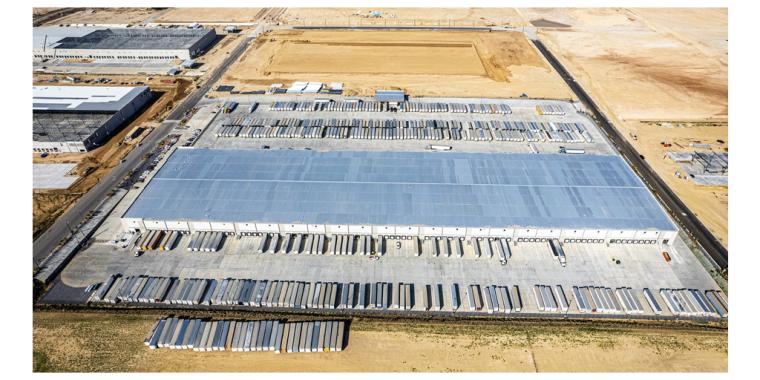This is an aerial photograph of a large industrial compound, primarily featuring a warehouse with various trailers and containers around it. The warehouse has a gray roof and off-white sides, and numerous dark blue, dark gray, and off-white tractor trailers are either docked or waiting to dock. The area surrounding the warehouse is light beige, suggesting it could be dirt or farmland, with no trees or grass visible. Roads flank both sides of the warehouse, with additional buildings located in the upper left corner of the image. A parking lot with cars is situated on the left side of the main building. This scene captures a storage or cargo area, where the main warehouse appears to be central to operations, with multiple trailers actively involved in loading and unloading goods.